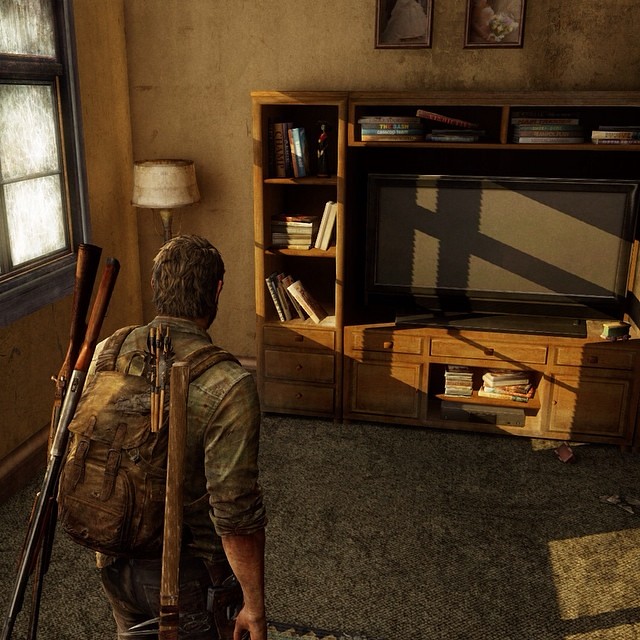In this square image, likely from a video game or an illustrated picture, we see a muted, somewhat dark scene dominated by earthy tones such as browns, camouflage greens, and beiges. The foreground features the back of a man positioned in the lower left corner, visible from the thigh up. He is dressed in army camouflage attire, with his long-sleeve shirt rolled up to the elbows. Strapped to his back are two rifles housed in a holster, as well as a backpack that matches the army fatigue colors. Additionally, a long mallet with a sharp black edge dangles off his right side. The man has dark brown hair, partially covering his ears, and his lighter skin tone is visible. Ahead of him, in a darkened room, stands a large open bookcase wall unit that also features a flat-screen TV. The scene, with its muted colors and detailed composition, evokes a sense of rugged readiness and anticipation.